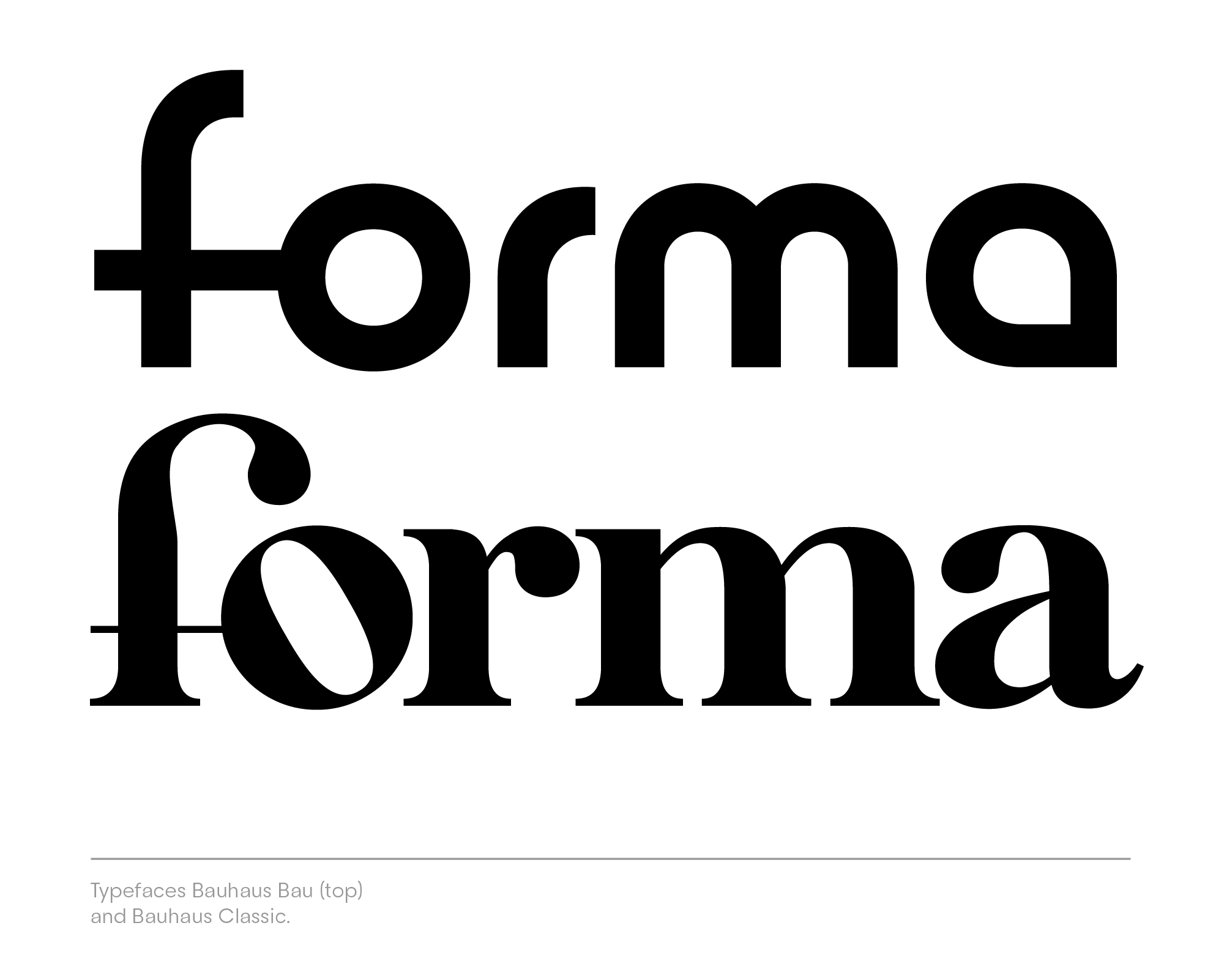This image showcases two different typefaces presented against a completely white background. At the top, the word "Forma" is displayed in a large, black, playful font. In this font, the 'F' and 'O' are creatively connected by the crossbar of the 'F', and both the 'F' and 'R' have partially drawn segments, giving them a futuristic look. The 'R' has a short nose, the 'M' is symmetrical, and the 'A' resembles a circle with a diagonal teardrop shape to the right, while still being identifiable as an 'A'. Below this, the word "Forma" appears again in a different, more traditional font. Here, the 'F' is fully formed with a subtle connection to the slightly tilted 'O'. The 'R' is complete, the 'M' is stylized, and the 'A' follows conventional design. Beneath these two words is a thin gray line, followed by a line of text at the very bottom left of the image that reads: "Typefaces Bauhaus, Bau Top, and Bauhaus Classic." These descriptions highlight the contrast between the two typefaces, showcasing their unique characteristics and stylistic differences.